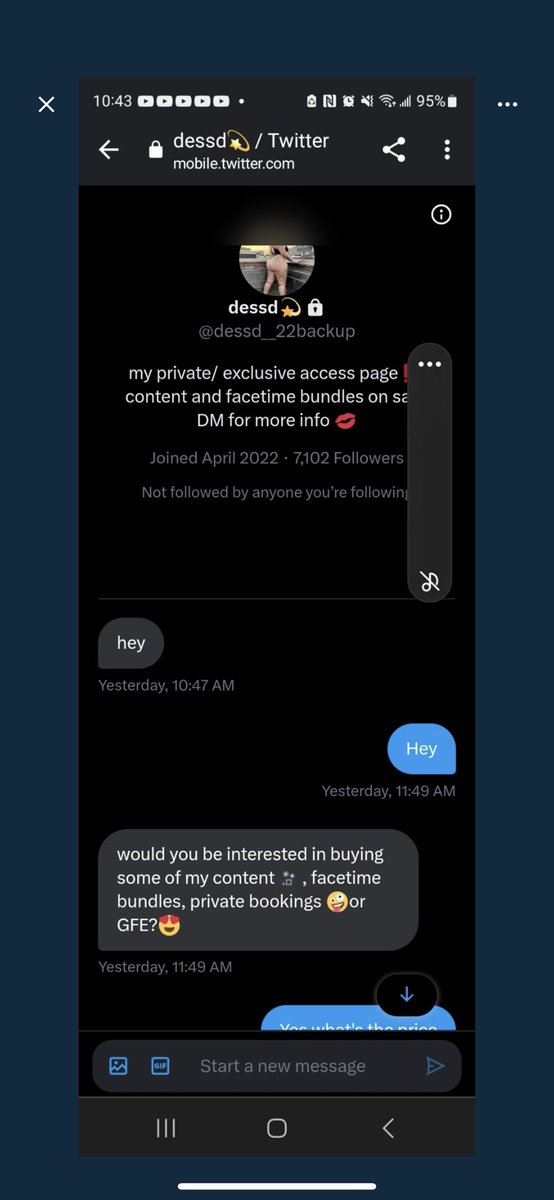**Screenshot Description from Twitter Profile:**

At the top of the screenshot, a profile picture of a girl is visible, although her face is not shown. She is holding onto a rail, wearing a black shirt and pink shorts or hot pants, with her legs slightly spread apart. Her username is "dessd," accompanied by a shooting star emoji. Her profile is marked as private.

- **Profile Information:**
  - **Username:** dessd ✨
  - **Handle:** dessd__22 (backup account)
  - **Profile Lock Status:** Private (indicated by a lock icon)
  - **Color Scheme:** Username and lock icon are in white; handle is in gray

- **Tweet Content:**
  - **Message:** "My private/exclusive access page! ❗️ Content and FaceTime bundles on sale. DM me for more info 💋"
  - **Date Joined:** April 2022
  - **Followers:** 7,102
  - **Following Status:** Not followed by anyone you're following
  - **Background:** Dark mode (black background)
  - **Text Color:** Dessd's messages in gray speech bubbles; other user's messages in blue speech bubbles

- **Message Exchange:**
  - **Dessd:** "Hey"
  - **Other Person:** "Hey"
  - **Dessd:** "Would you be interested in buying some of my content? There are video camera FaceTime bundles, private bookings, and GFE (girlfriend experience) 💓."
  - **Last Message Time:** 11:49 AM
  - **Unread Response:** First word visible is "You"

- **Message Input Bar:**
  - **Text:** "Start a new message" in gray
  - **Icons:** Blue icons for picture uploads, GIFs, and sending messages

- **Bottom Navigation:**
  - **Gray Line Icons:** Three gray lines, the square home button, and the gray back button

Overall, the screenshot exhibits a private Twitter account promoting exclusive content and services through direct messages, emphasizing the profile's dark theme and detailed interface elements.